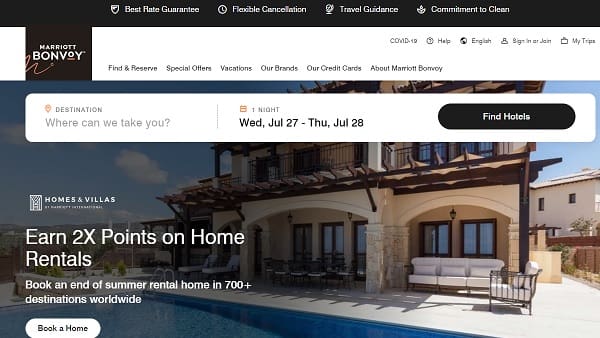The screenshot captures the main page of the Marriott Bonvoy hotel chain website. The top center of the page features a black horizontal bar displaying links labeled "Best Rate Guarantee," "Flexible Cancellation," "Travel Guidance," and "Commitment to Clean," providing crucial information for users. The Marriott Bonvoy logo, in white text on a dark brown background, is positioned at the top left corner.

Dominating the center of the page is a prominent white search bar where users can input their trip details to find hotels. The left side of this bar prompts users with "Destination. Where can we take you?" allowing them to enter a city or specific hotel. The center of the bar indicates a potential booking with the text, "One night, Wednesday, July 27th to Thursday, July 28th," clickable to open a calendar for selecting different dates. 

On the right-hand side of the search bar, a dark green box with white text reads "Find Hotels," which users can click after entering their destination and timeframe to proceed with their search.

The website's background showcases an upscale hotel with a luxurious pool in the foreground. At the bottom left, white text advertises, "Earn 2x points on home rentals. Book an end of summer rental home in 700+ destinations worldwide," highlighting Marriott's home rental options. A white button labeled "Book a Home" in the bottom left corner allows users to opt for a home rental instead of a traditional hotel stay.